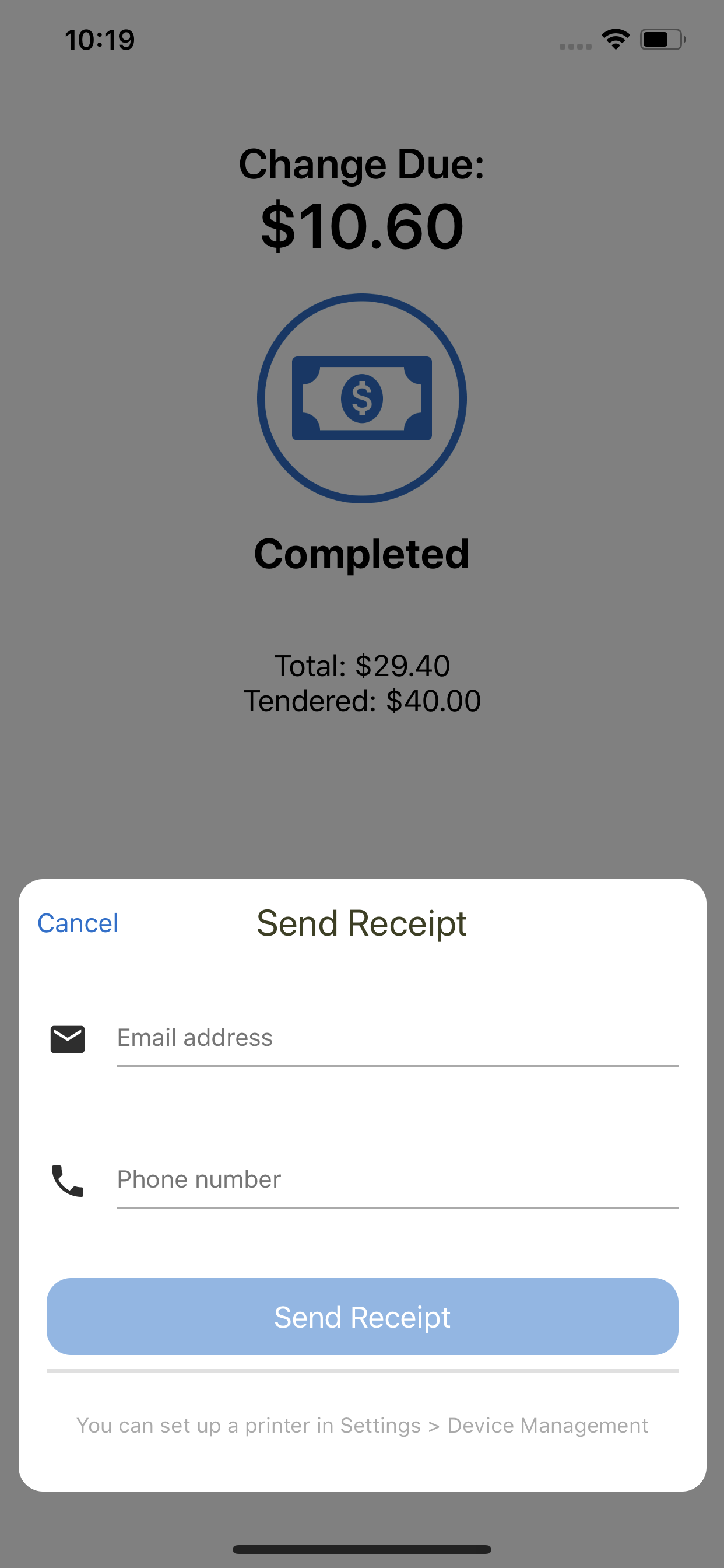This is a detailed screenshot of a cell phone displaying a transaction completion screen against a gray background. At the top of the screen, the time reads 10:19. There are four signal strength dots on the right side, indicating a strong connection to Wi-Fi, and the battery icon shows it is slightly more than half full.

The main content of the screenshot focuses on the transaction details. At the very top, the phrase "Change Due" is displayed, followed by the amount $10.60. Below this, a circular icon contains a rectangle with a dollar sign, representing money. Directly beneath, the word "Completed" is shown in black text.

Further down, the transaction breakdown lists "Total: $29.40" and "Tendered: $40.00". There is an option to send a receipt, with fields to input an email address or phone number. A clickable blue line labeled "Send Receipt" facilitates this action. To the left, a "Cancel" button is also present.

At the bottom, additional options are provided to set up a printer and access device management settings. This screenshot is a typical example of what a customer might see on their phone after making a payment and choosing to receive an electronic receipt instead of a paper one. The screen confirms that the payment is complete and provides all necessary information to send the receipt either via email or phone.